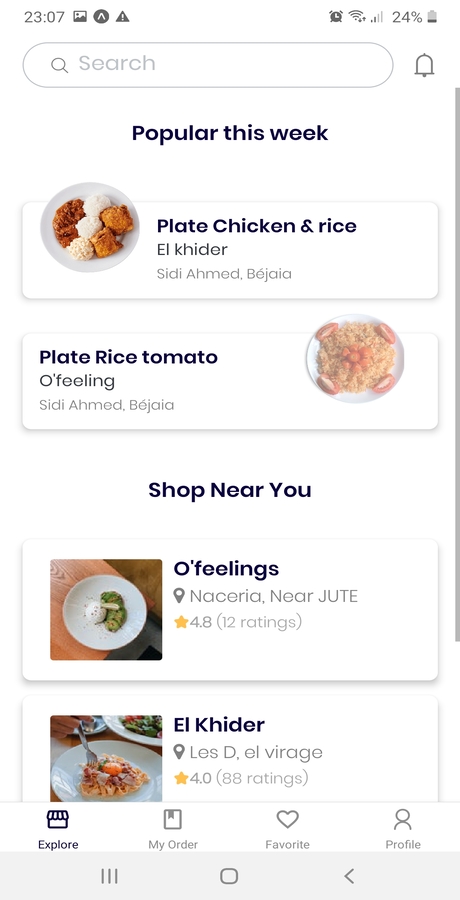The screenshot showcases an interface of an online food ordering platform, possibly an app where users can order from different restaurants. At the top of the interface, there is a search bar with the time displayed as 23:07. The top bar also features various icons including a photo icon, a navigation icon, an alert icon, an alarm icon, the WiFi signal strength icon (showing 2 out of 4 bars), and a battery icon indicating 24% remaining. 

Directly below the search field, there's a bell icon followed by the text "Popular this week." The interface displays food items with photographs in rectangular floating panels that have a slight drop shadow for a 3D effect. 

The first item is labeled "Plate Chicken and Rice," by Sidi Ahmed Bashai, featuring a high-quality photograph of the dish. It is followed by another item labeled "Plate Rice, Tomato, Oh Feelings" by Sidi Ahmed Bashai.

Further down, there's a section labeled "Shop near you," displaying another plate of food titled "Oh Feelings," from Nasiriyah near Jute, rated 4.8 based on 12 ratings. Each listing includes a star rating and a map icon for location details.

Additionally, there's information about "Less D and L Viraj," showing a rating of 4.0 based on 88 ratings. On the right side of the screen, a long gray scroll bar is visible, indicating more items can be viewed by scrolling.

At the bottom of the interface, navigation options are displayed: "Explore," "My Order," "Favorites," and "Profile."